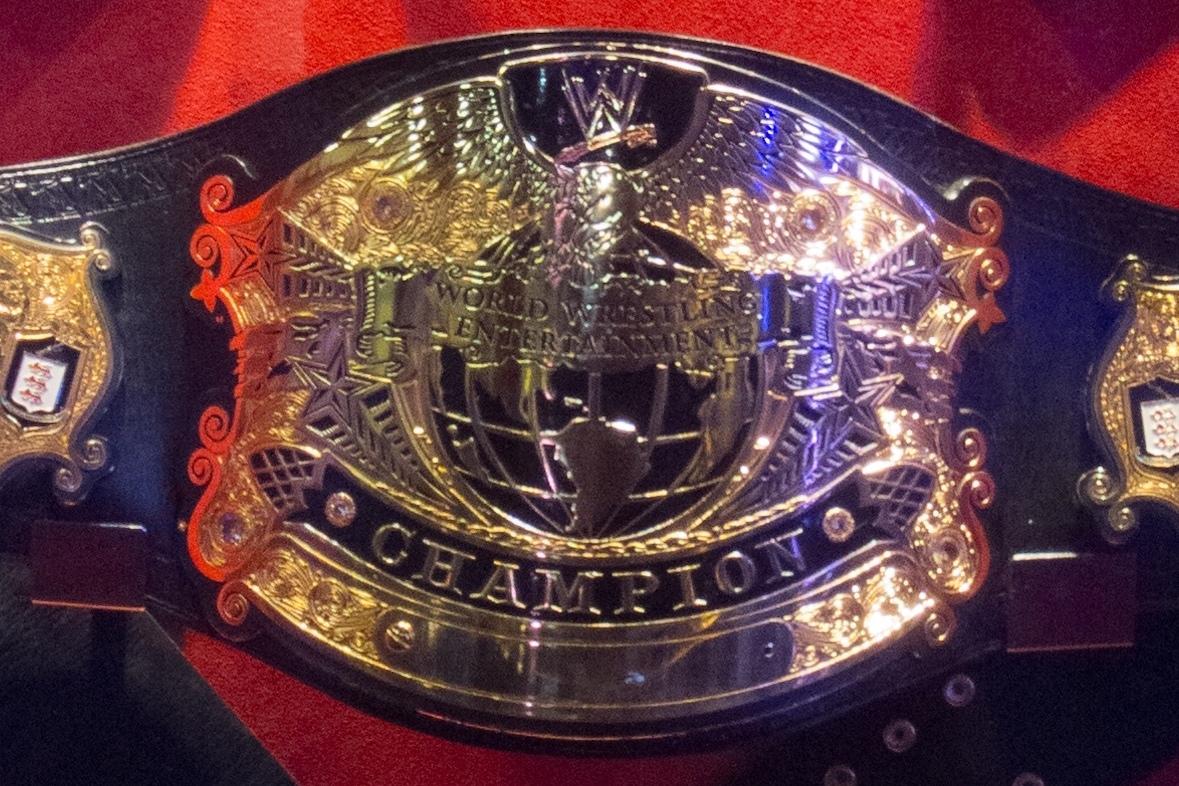This is an up-close photograph of a WWE World Wrestling Entertainment championship belt. The belt is prominently displayed, sitting on a stand against a backdrop that transitions from red at the top to black at the bottom. The main buckle of the belt features an intricate, large gold emblem with silver and black accents. At the very top is the iconic W logo, resembling two stacked W's. Beneath the logo, two large wings extend upward, enclosed within the elaborate gold emblem. Below the wings lies a globe, topped by a ribbon-like gold banner. Underneath this globe, a large black ribbon with raised gold lettering spells out "Champion." Flanking the central buckle on both sides are two equally ornate, smaller gold metal pieces, contributing to the grandeur of the belt. The belt itself is made of black leather, adding a stark contrast to the metallic details.